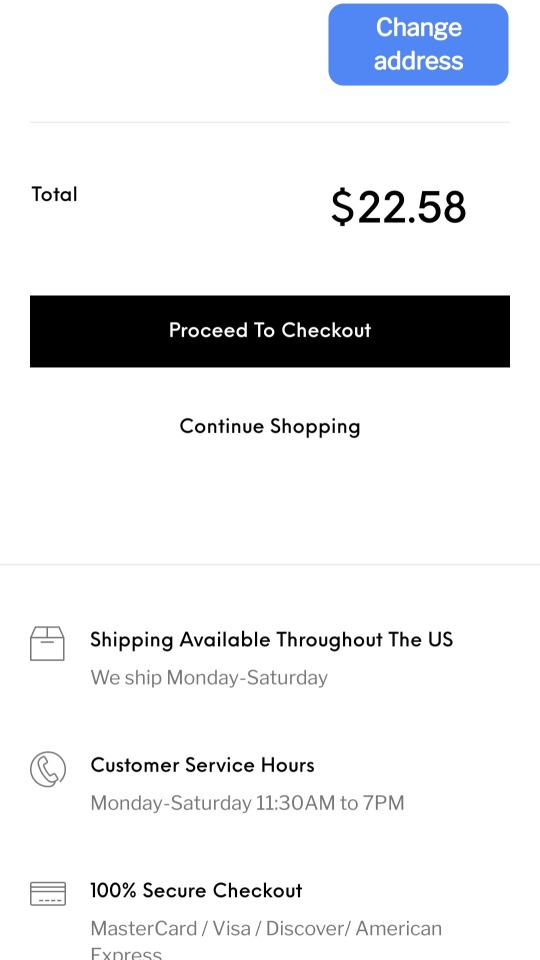The image shows a smartphone screen displaying a webpage on a completely white background. At the top, there is a small blue box with white text that reads "Change Address." Below this, the total amount is displayed in black lettering: "Total: $2258." Directly beneath this amount is a black button labeled "Proceed to Checkout," and below that, there is a link that says "Continue Shopping."

Further down the screen, an informative section begins with a black pocketbook icon next to the text: "Shipping available throughout the US. We ship Monday through Saturday." The next line features a phone icon followed by "Customer Service Hours" and states, "Monday through Saturday, 11:30 a.m. to 7 p.m." Another section emphasizes "100% Secure Checkout" with a credit card icon, listing accepted payment methods: MasterCard, Visa, Discover, and American Express.

The webpage does not specify the company name or the item being purchased, suggesting this is likely the second screen that appears after an item has been added to the shopping cart.